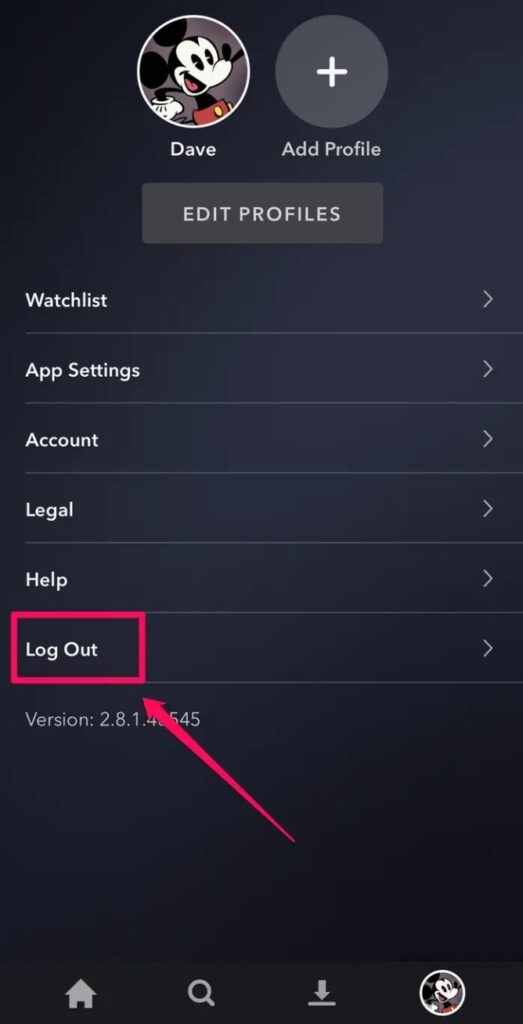This image is a detailed screenshot from a mobile device, displayed in portrait orientation against a dark, blackish-blue background. At the top of the screen are two circular icons. The left circle, bordered in white, features an image of Mickey Mouse and the name "Dave" beneath it in white font. The right circle is gray with a white plus sign and the label "Add Profile" beneath it.

Below these icons, there is a rectangular gray button labeled "Edit Profiles" in white font. Further down the screen, a series of menu options are listed, each separated by a thin gray horizontal line. These options include "Watch List," "App Settings," "Account," "Legal," "Help," and "Logout," all written in white font with right-facing gray arrows next to them.

At the bottom of the screen, it reads "Version 2.8.1.4," followed by an obstructed number, "545." The "Logout" option is prominently highlighted with a bright reddish-pink rectangular box surrounding it. Additionally, a red arrow pointing upward and to the left directs attention towards the "Logout" box, indicating that it might be an instruction or prompt to click on it.